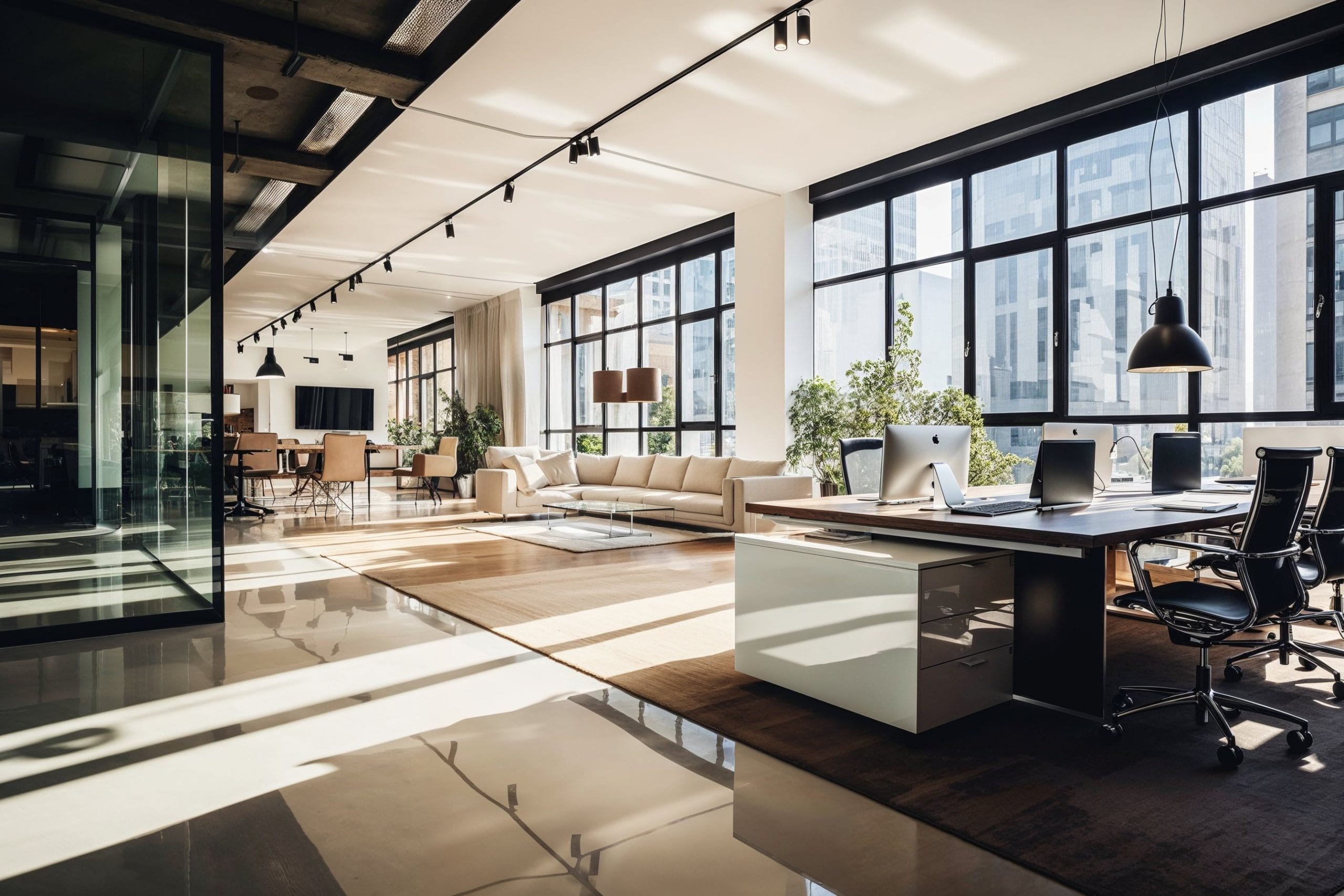This image showcases a spacious and modern loft-style office situated within a city high-rise, characterized by its expansive use of windows that offer sweeping views of downtown skyscrapers. The front of the space is predominantly lined with large, black-framed windows, flooding the interior with natural light and casting dynamic shadows on the polished tile floor. The decor is a sleek mix of white and black, featuring a white ceiling with a black track lighting system that runs along its length. 

On the left, an inviting lounge area is arranged with a white sectional couch, a glass coffee table, and a small white rug, providing a comfortable spot for relaxation or informal meetings. Moving towards the center, a more structured space emerges with a desk adorned with multiple computer screens, laptops, and a white computer base, situated against white columns. This desk is paired with several black chairs, suggesting a collaborative work environment.

In the mid-ground, an elegant dining or conference area is marked by a brown table with tan chairs around it, hinting at versatility between casual dining and formal meetings. This area is further defined by its proximity to an adjacent glass wall, which appears to lead into another room, adding to the openness of the loft. The overall aesthetic is punctuated by black details, such as a black desk, black windows, and a sleek black lamp overhead, all harmoniously integrated into the predominantly white furnishings with subtle black trims.

Rays of sunshine penetrate the loft, particularly highlighting a pathway from the bottom left to the center of the room, emphasizing the airy and bright atmosphere of this sophisticated, urban office space.